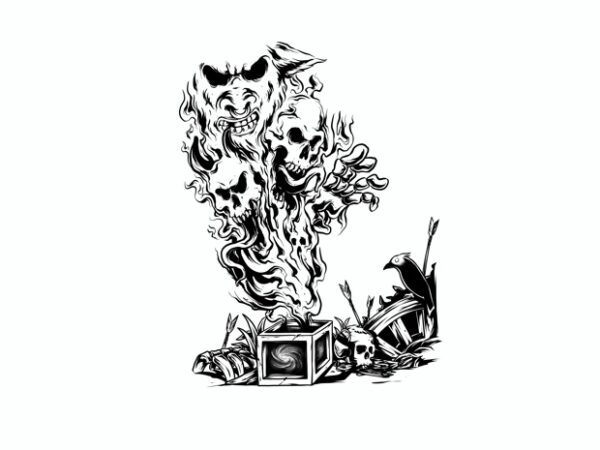This intricate black-and-white drawing, rich in detail despite its small size, depicts a grim, haunting scene. At the center left, a cube with spiral patterns on two of its faces sits on the ground. Emerging from its open top is a swirling plume of smoke, transforming into various ghastly faces. Two of these faces are skeletal, one with prominent horns and a protruding tongue, while another appears ghostly. Ascending further, a demonic, bull-like face with a sneering expression and a bull ring dominates the upper part of the smoke. Intertwined within the smoke is a skeletal hand, extending ominously. On the ground, several arrows penetrate the earth, accompanied by a scattered rib cage and a skull with arrows lodged in it. Toward the bottom right, a black bird, appearing raven-like with white eyes, perches on the remnants of a broken wheel. The scene conveys a sense of dark magic and eerie foreboding, with the background artfully rendered in stark white to emphasize the macabre details.